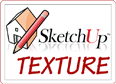This is an extremely close-up image of a weathered wooden shingled roof. The shingles, or shakes, are predominantly ash-colored, hinting at significant exposure to the elements, and they vary in size, including longer, shorter, wider, and thinner pieces. Some shingles appear darker, possibly due to aging, oil spills, or some other type of gunk, with noticeable black spots, particularly on the right side. Several shingles are cracking at the ends, which further emphasizes their age. The photograph reveals a large section of the roof, showing at least two dozen rows of tightly packed wooden shakes, all seemingly intact. Dominating the center of the image is a barely readable white circular watermark. This circle contains an illustration of a house with a pencil beside it, and there's likely additional text around and across the circle, although the letters are too faint to decipher against the weathered background.